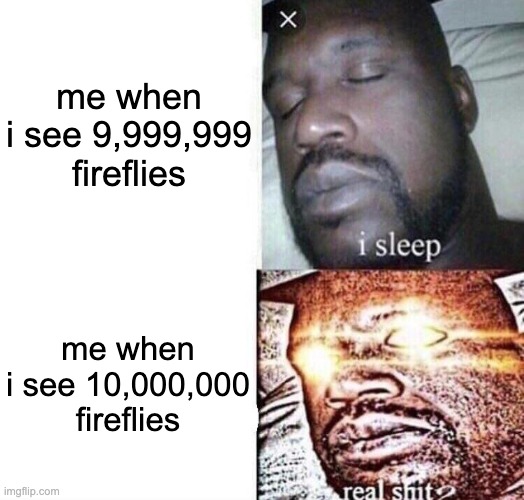A detailed caption for the described meme could be:

"This meme features a humorous juxtaposition of two images of Shaquille O'Neal to convey a comedic reaction to different quantities of fireflies. The layout consists of two vertically stacked sections, each with text and an accompanying image. 

In the top section, the text on the left, set in black on a white background, reads: 'Me when I see 9,999,999 fireflies.' To the right is an image of Shaquille O'Neal asleep, with the overlay text 'I sleep' in white just above his head. Additionally, a black circle with an 'X' is superimposed on the top-right corner of this picture, resembling a closed internet tab element. 

The bottom section text says: 'Me when I see 10,000 fireflies.' The corresponding image again features Shaquille O'Neal, but this time heavily edited with glowing yellow eyes and radiating yellow lines, giving him a dramatic, energized look. The overlay text in this image is in white and reads: 'Real shit.' The meme is watermarked with 'imgflip.com' in gray text at the lower left corner, indicating the platform where it was created or shared."

This descriptive caption thoroughly explains each element of the meme, providing a vivid image for anyone who has not seen it.